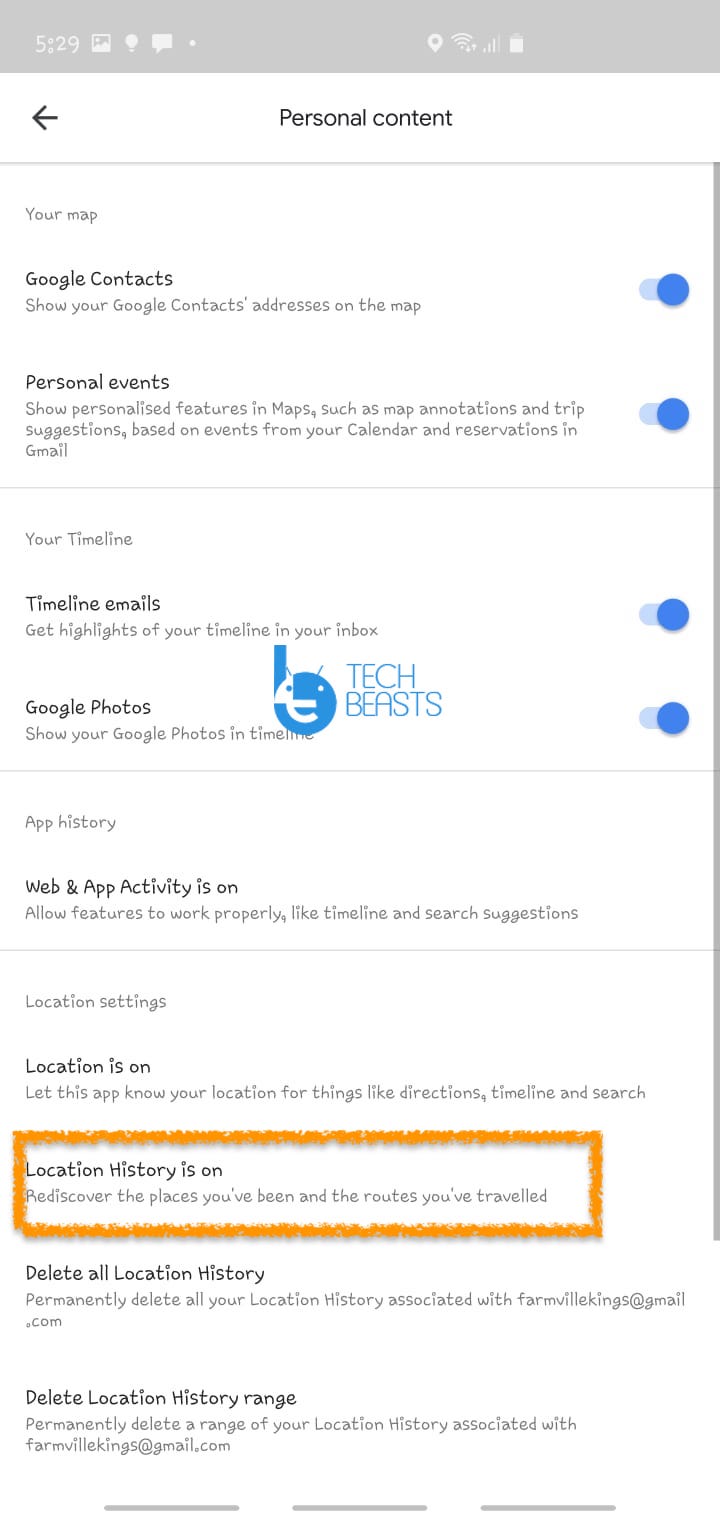A detailed depiction of a user interface screenshot:

The image, labeled as "Texted 529," provides a comprehensive view of several app features and settings. Prominent elements include an illuminated lightbulb icon adjacent to a comment bubble inscribed with "pin." The screenshot displays symbols for full Wi-Fi connectivity and battery status. A leftward arrow signifies navigation to previous content. 

Located in the "Personal Content" section, a line map reveals key features:
- "Show your Google Contacts' Addresses on the Map," highlighted with a blue tunnel effect, which denotes an enhancement layer.
- "Personal Events" option enables map annotations and trip suggestions, tailored based on calendar events, reservations, and Gmail data.
- "Your Timeline" aggregates and highlights inbox activity, leveraging Google Photos to display images and chronicle history.

The "App History and Web Activity" feature, marked as active, permits optimized functionality such as timeline searches and suggestion accuracy. Users are prompted to allow the application to access location data for precise direction inside the app.

An orange border indicates active "Location History," which lets users rediscover visited places and traveled routes. There are options to delete all location history:
- A command to permanently erase all location records associated with a user’s Google account (example: fireorvolcano@gmail.com).
- Another option provides granular control to delete location history within a specific range for the same account.

The overall layout is user-centric, integrating personalized features and seamless connectivity to enhance navigation and data management experience.